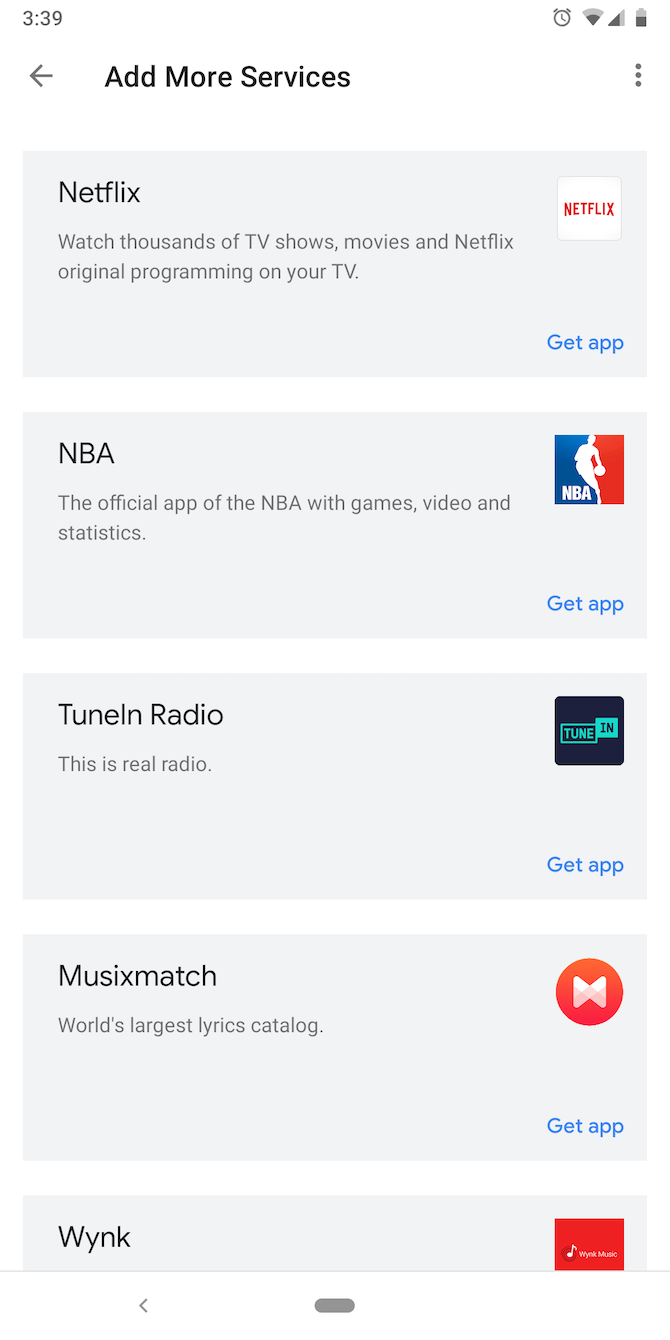The image is a screenshot of a cell phone displaying a "Services" page within an application. The screen's top center features the text "Add More Services" in black, indicating the purpose of the page, with various app links available for addition to the cell phone. At the top left corner, the phone's current time is displayed as 3:39, while the top right corner includes standard status icons for data connection, cell signal strength, and battery life.

Below the header, there is a left-facing gray arrow, positioned left of the "Add More Services" text, allowing users to return to the previous page in the application. Further down, five horizontal gray boxes showcase different apps available for download: Netflix, NBA, TuneIn Radio, Musixmatch (spelled M-U-S-I-X-M-A-T-C-H), and Wink (spelled W-N-Y-K). Each box contains a brief description of the respective app, alongside the app's logo positioned at the top right corner of the box. In the bottom right corner of each gray box, the text "Get App" appears in blue, serving as a clickable link that directs users to the App Store to download the selected application.